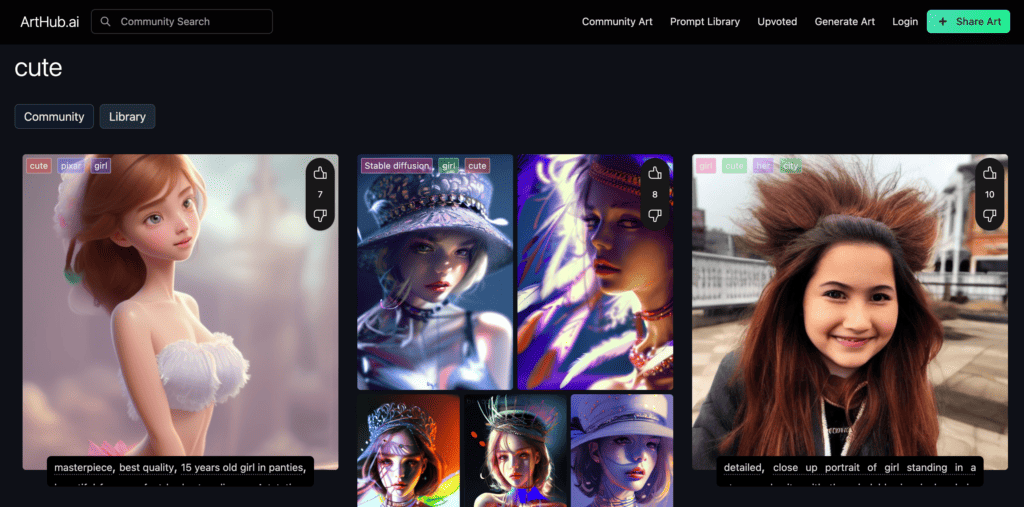The image features a screenshot of a website named ArtHub.ai, set against a black background. In the upper left corner of the screenshot, the text "ArtHub.ai" is prominently displayed in white. Immediately to the right, the phrase "Community Search" is visible. On the far right side are several buttons in white text, listed from left to right: "Community Art," "Prompt Library," "Upvoted," "Generate Art," and "Login." Additionally, there is a green button with black text that reads "Share Art" next to a plus (+) symbol.

Dominating the left side of the screenshot is the large text "Cute." Below this header is a visual showcase from the image library. The first image on the left is a digital illustration of a Disney-like girl with red hair, wearing a white bikini top. Next to this illustration, there is a square grid containing five images of young women, each adorned in a different style of hat. To the right of this grid is a life-like photo featuring a girl with her hair standing straight up, set against a realistic background.